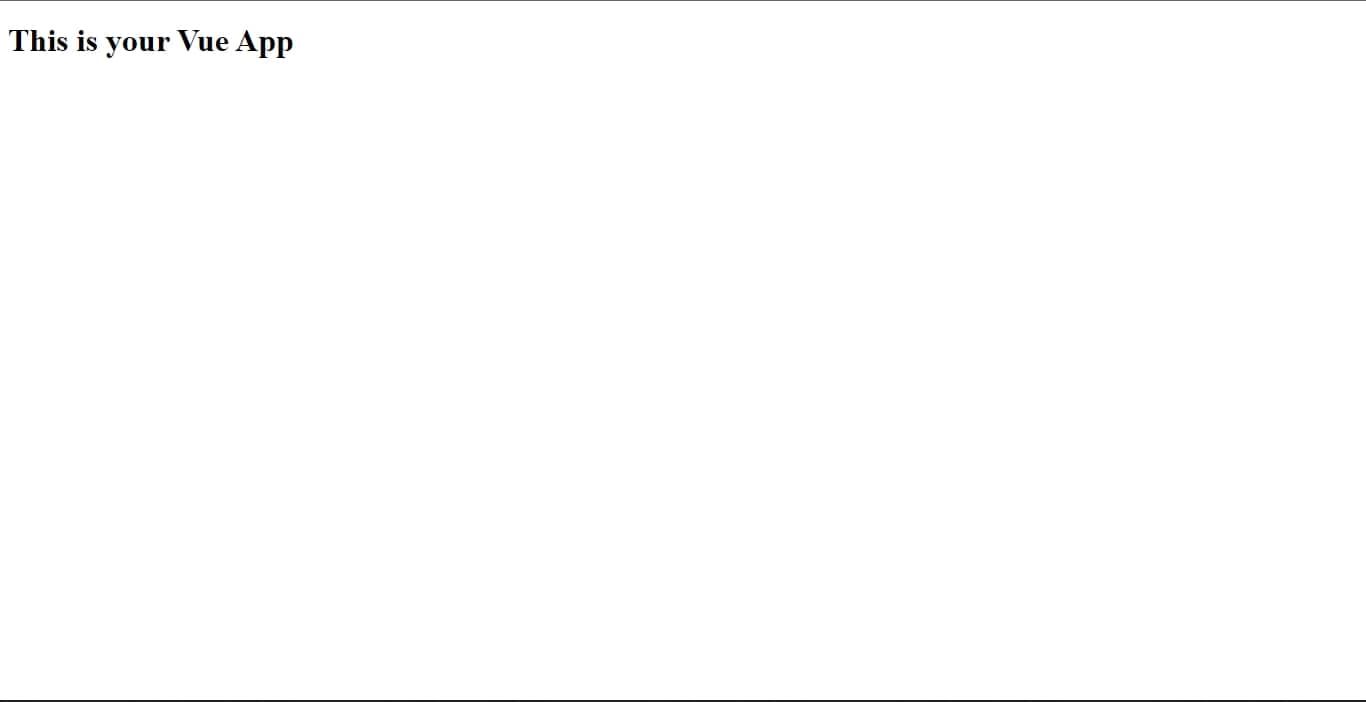A minimalistic application interface is displayed on a stark white background. The design is framed by two thin, horizontal black lines—one at the top and one at the bottom of the screen. In the upper left corner beneath the top line, there is black text in a font resembling Times New Roman that reads, "This is your VIEW app." The capitalizations are precise, with the 'V' in 'VIEW' and the 'A' in 'app' both distinctly capitalized. The remainder of the screen is entirely white, devoid of any additional content or context, suggesting either a placeholder interface or a potential issue with the application's content loading.